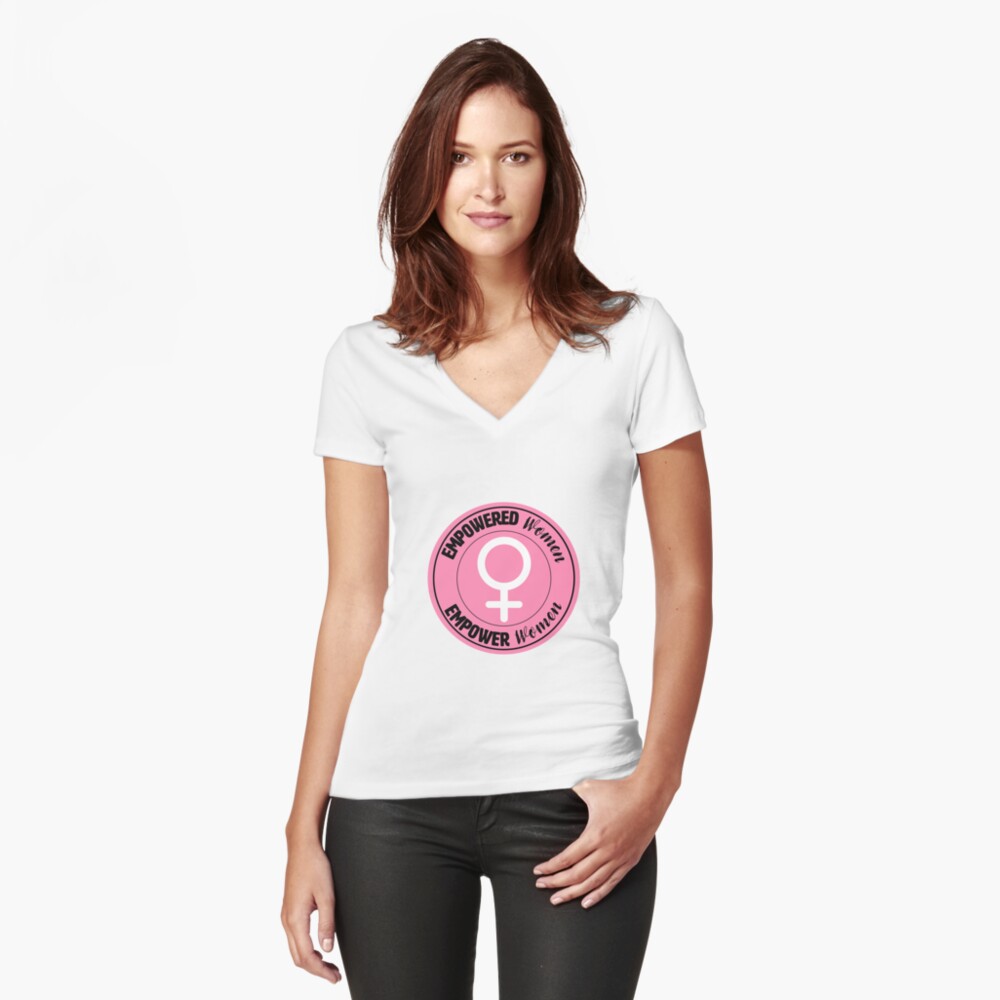The image is a stock photo of a young woman in her early 20s, likely a model, standing against a plain white background. She is depicted from her thighs up, showcasing her long, slender arms and tall, lean figure. She has a light complexion and shoulder-length, slightly waved brunette hair. Her makeup is minimal, with light pink lipstick emphasizing her features.

The woman is wearing a close-fitting, white, V-neck, short-sleeved shirt tucked into her black skinny jeans, with one thumb casually hooked into the waistband of her pants while her other hand rests at her side. Prominently displayed on the front of her shirt is a circular pink emblem with a white female symbol (a circle with a cross beneath it) in the center. Surrounding the symbol, in bold black text, are the phrases "Empowered Women" on the top half of the circle and "Empower Women" on the bottom half, underscoring the theme of female empowerment.